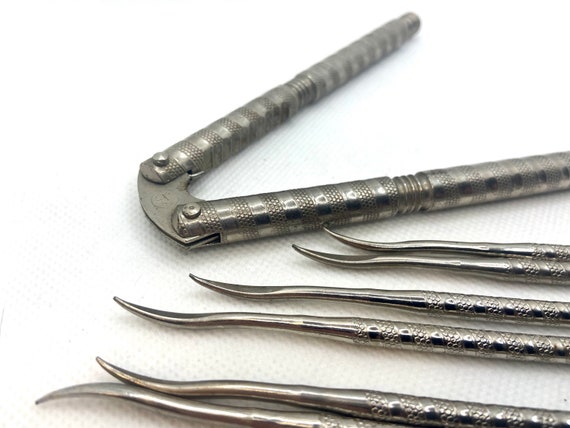The image features an array of seven brushed metal tools displayed on a white, slightly textured paper towel, reminiscent of those used in dental offices. Central to the image is an old-fashioned handheld nutcracker, identifiable by its two prong-like mechanisms for cracking walnuts or possibly crabs. This nutcracker, characterized by its two bolt hinges and ergonomic design for hand grip, appears predominantly open and is more grayish in color rather than shiny silver. Surrounding it are six additional metal instruments, each resembling long picks with narrow, slightly curved cupped edges at the top. These tools also display a striped texture along their bodies. Though their exact function is unclear, their design suggests they could be used for prying or digging. All tools share a consistent brushed metal finish, providing a cohesive visual theme.